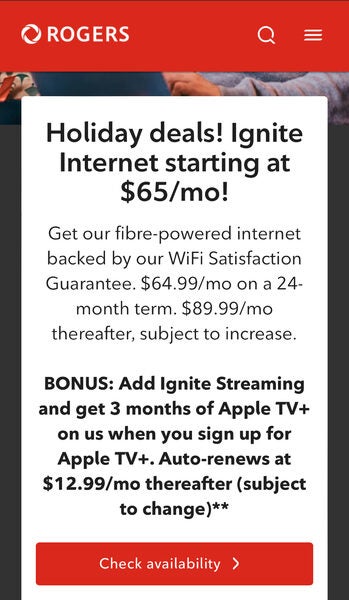The image is a screenshot of a mobile phone displaying a promotional offer from Rogers. At the top of the screen, set against a red background, is a circular braided rope logo accompanied by the text "Rogers." Adjacent to the logo, there's a magnifying glass icon for search functionality and a menu icon, represented by three horizontal bars, for additional options.

Prominently featured in the center is a white box with bold black text that reads: "Holiday Deals: Ignite Internet starting at $65 a month." Below this bold header, in regular black font, the offer elaborates: "Get our fiber-powered internet backed by our Wi-Fi satisfaction guarantee $64.99 a month on a 24-month term. $89.99 a month thereafter, subject to increase." 

Additionally, a bonus offer is mentioned: "Add Ignite Streaming and get three months of Apple TV Plus on us when you sign up for Apple TV Plus. Auto-renews at $12.99 a month thereafter. Check availability, subject to change."

At the bottom of the screen, there is a conspicuous red button labeled "Check Availability."

In the background, behind the promotional text, faint outlines of people's hands or arms can be discerned, adding a subtle layer of human presence to the image.